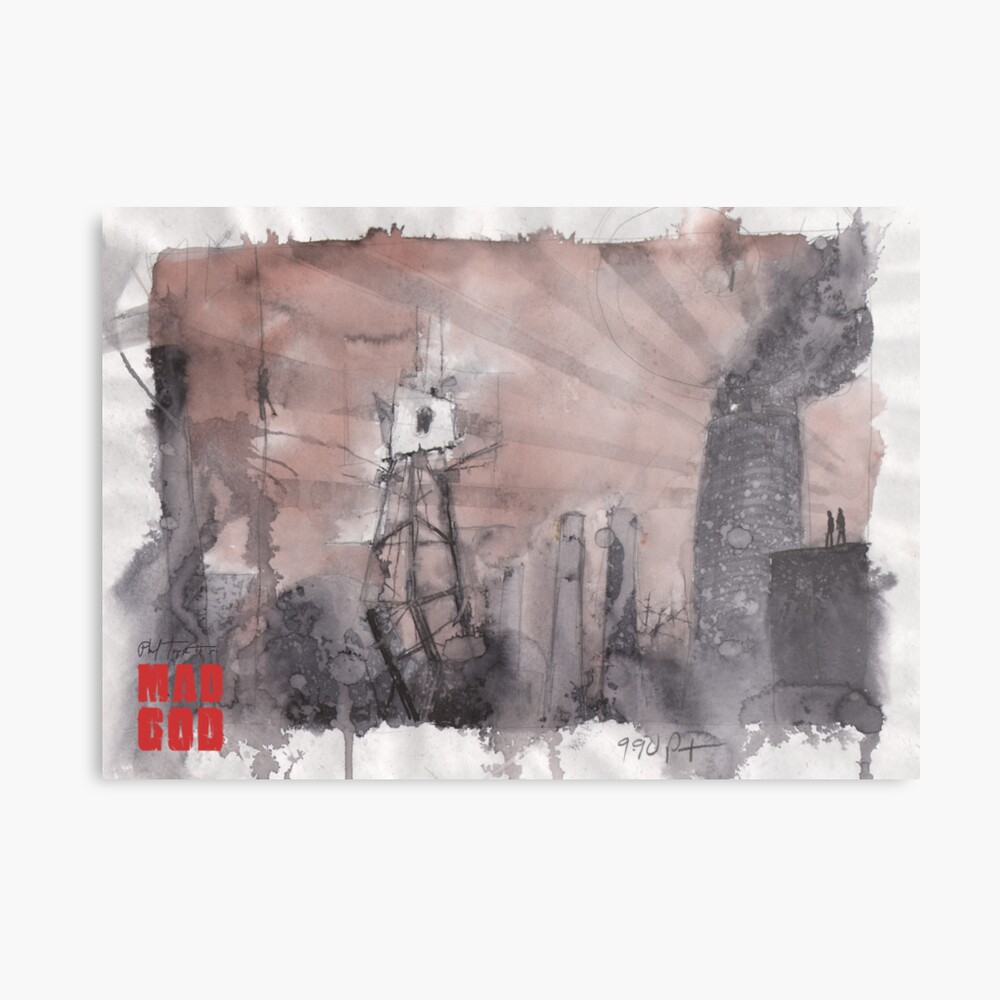The image prominently features the words "Mad God" in bold red letters at the bottom left corner, with a light gray background and a light brown interior section. The artwork appears to be a messy, surreal watercolor painting with a mix of gray, tan, and brown hues. The composition includes a large, collapsing silver tower supporting a small structure, with heavy smoke billowing from smokestacks. Rays of gray light emerge from the right side, while a black wiry frame is present in the background. On the left side, there is a long vertical rope with the silhouette of a person descending it. Additionally, there are two silhouettes of people standing off in the distance on the right side. The painting has an unstable, almost dripping appearance as if water has smudged the colors, contributing to its chaotic and surreal aesthetic.